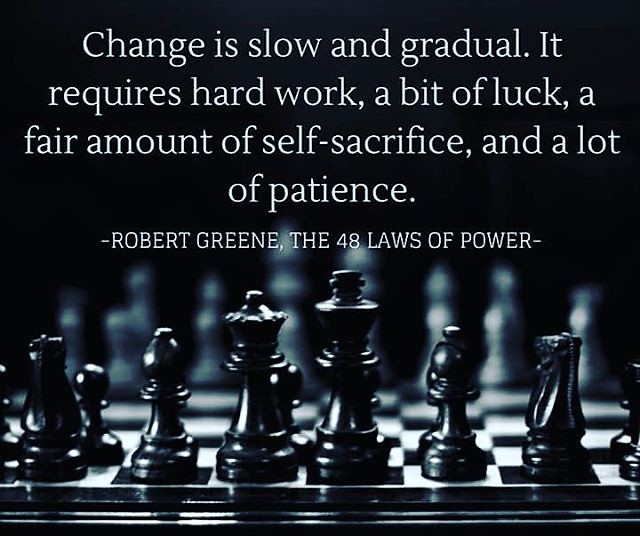The image is a motivational poster with a black background, dominated by white centered text in a large font at the top half. The text reads: "Change is slow and gradual. It requires hard work, a bit of luck, a fair amount of self-sacrifice, and a lot of patience." Below this quote, attributed to Robert Greene from "The 48 Laws of Power," are details such as two minus signs framing his name and the book title. The bottom half features an intricate black-and-white chessboard in the foreground, with the black chess pieces set up neatly in their initial positions, facing the viewer. In the hazy background, the white chess pieces are also positioned at the start of the game, creating a sense of depth and transition.